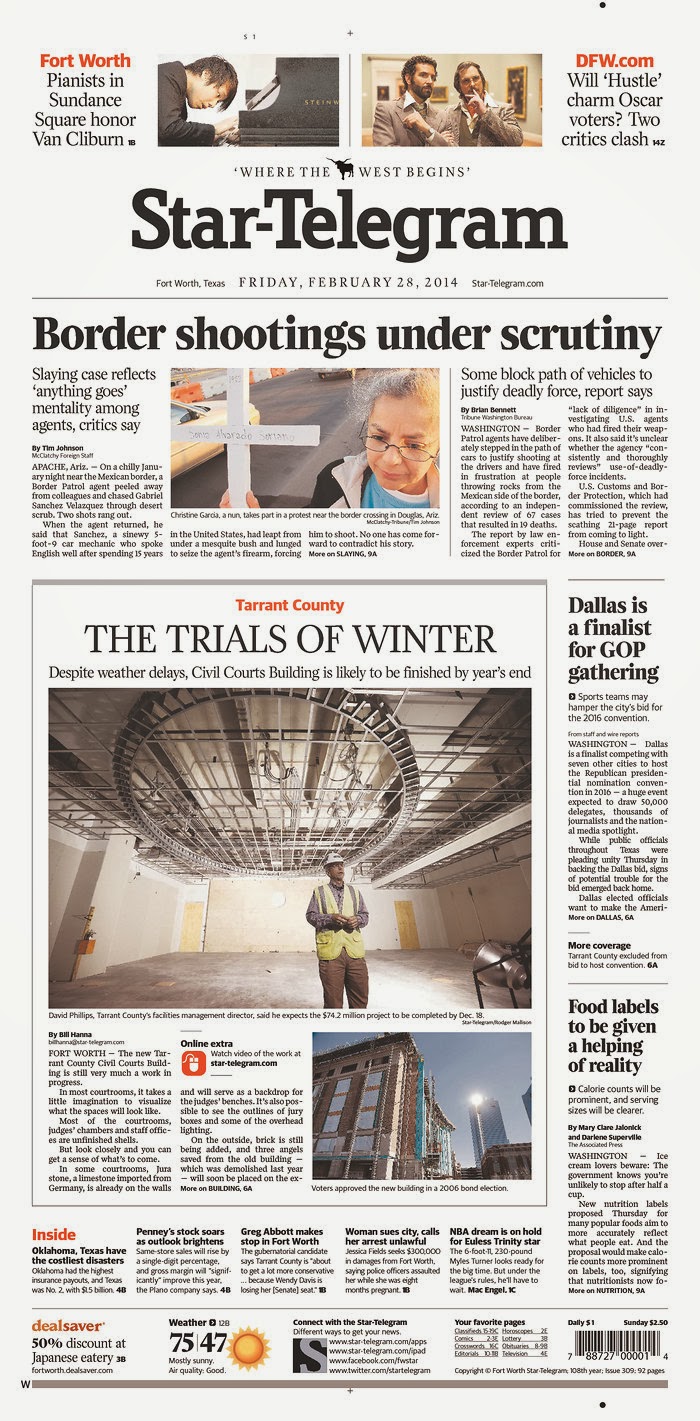This is a vertically-oriented, rectangular image of the front page of a newspaper. Dominating the upper portion is the newspaper's name in bold, black font: *Star-Telegram*. Above the title, the slogan "Where the West Begins" is prominently displayed. Just beneath the newspaper’s name, the issue date is mentioned, though it is not clearly readable.

At the top of the page, there are two horizontally-aligned rectangular photos. The left photo features a man playing a piano, facing the right edge of the image. Adjacent to this photo is a headline in red and black fonts: *Fort Worth Pianist in Sundance Square Honor Van Cliburn.* The right photo has a text overlay in bold red font: *DFW.com*. Below the red letters, in black font, it reads: *Will 'Hustle' Charm Oscar Voters? Two Critics Clash.*

Beneath the newspaper’s name and the date, the primary headline in bold, black font reads: *Border Shootings Under Scrutiny*. Below it, in regular black font, is a subheading: *Slaying Sparks Debate on Agents' Conduct, Critics Say*. To accompany this article, there is an image of a woman wearing glasses, holding what appears to be a white cross. 

To the right of this, another article begins with the headline: *Some Block Path of Vehicles,* though the rest of the text is unreadable.

Lower down the page is a large article under the headline: *Trials of Winter*. The subheading reads: *Despite Weather Delays, Civil Courts Building Likely to be Finished by Year’s End.* Above this article, in red text, is the phrase: *Tarrant County*, and an image shows a man within what looks like an unfinished building.

Further down, another bolded headline in black reads: *Dallas is Finalist for GOP Gathering*, with possibly more text under it.

Additionally, there is an article titled: *Food Labels to be Given a Helping of Reality*.

At the very bottom left, the word *Inside* appears in red, accompanied by the beginning of another article and five small excerpts of other articles with corresponding page numbers listed in bold black font. There is also a barcode situated at the lower right corner of the page. The rest of the surrounding text is too small to be legible.